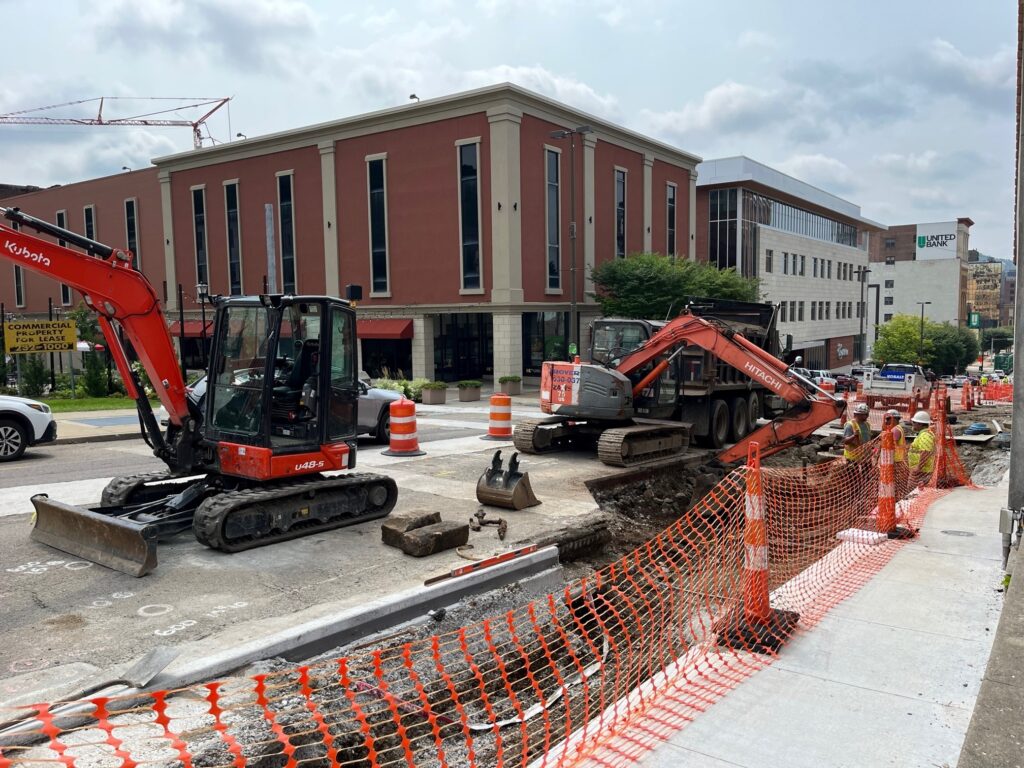The image captures a bustling construction site on a sunny day, showcasing two heavy-duty backhoes—black with red and orange parts, labeled Hitachi and Kubota—actively working on a section of a road. Along the bottom right of the photo, a red netted fence, supported by traffic cones, cordons off the area, indicating ongoing work. Nearby, workers wearing white helmets and high-visibility yellow vests manage the site, with some standing by a deep hole where one of the backhoes is excavating. Adjacent to this hole, a dump truck appears almost full with extracted material. The scene is lined by a sidewalk on the right, which is temporarily fenced off.

In the background, there are several buildings: a prominent red one with white pillars and elongated windows trimmed with white borders, followed by a glass-fronted brown building with a white roof and decorative brick facade. Further in the distance stands a structure marked with "United Bank" in bold letters, accompanied by a green icon. Cars are seen passing by on the road, and a sign on the left advertises commercial property for lease, with the phone number 232/100. Scattered clouds dot the blue sky, accentuating the vibrancy of the day.